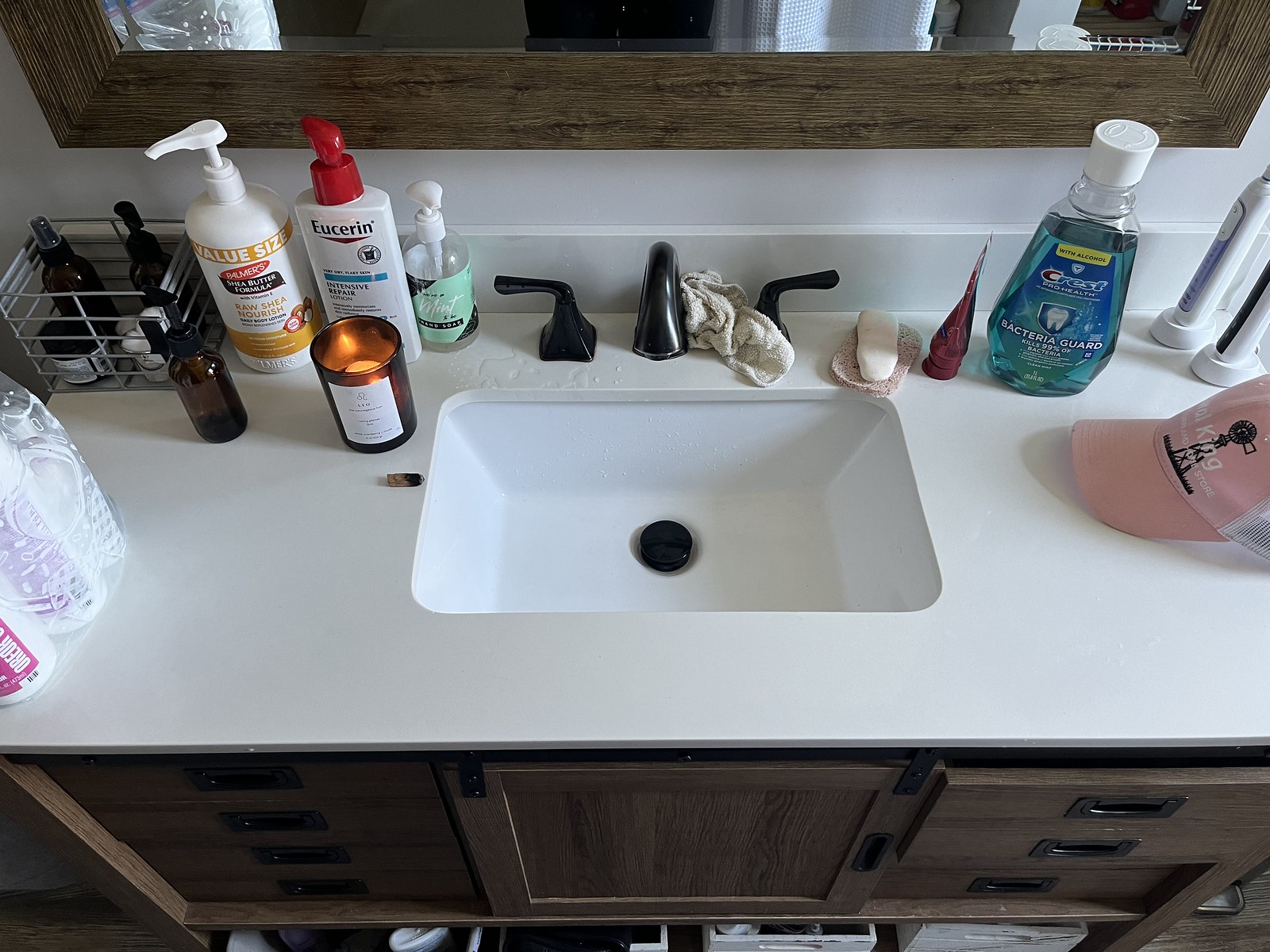In the image, taken in a bathroom during the day or under artificial light, the scene is bustling with details. The bottom of a mirror with a dark brown frame is partially visible in the background, along with the legs of the person taking the photo, who appears to be wearing black pants and pointing their camera down at the sink.

The sink is made of white marble or possibly white plastic, complemented by a black metal faucet and two black metal handles. On the far left, there is a small white metal basket containing various liquids, likely hair products. To the right of the basket, there are two white squirt bottles; one is a Eucerin bottle with a red cap, while the other is all white with gold writing that is difficult to read. Next to these bottles is a clear plastic hand soap dispenser with light blue, teal, and green accents.

In front of the dispenser, there is a votive candle in a golden yellow or stark brown holder, possibly lit. On the right faucet handle, a crumpled white cloth is draped. Next to the cloth is a white bar of soap, flanked by a small, unidentified pink bottle. Further right is a bottle of blue Crest mouthwash placed beside two mechanical toothbrushes, each sitting in a white and blue charging station. One toothbrush is white and black while the other is white and blue.

Lastly, a pink hat with an old-style windmill design is partially visible. The vanity area features multiple drawers on both sides with a large central door, all in a darker oak finish.